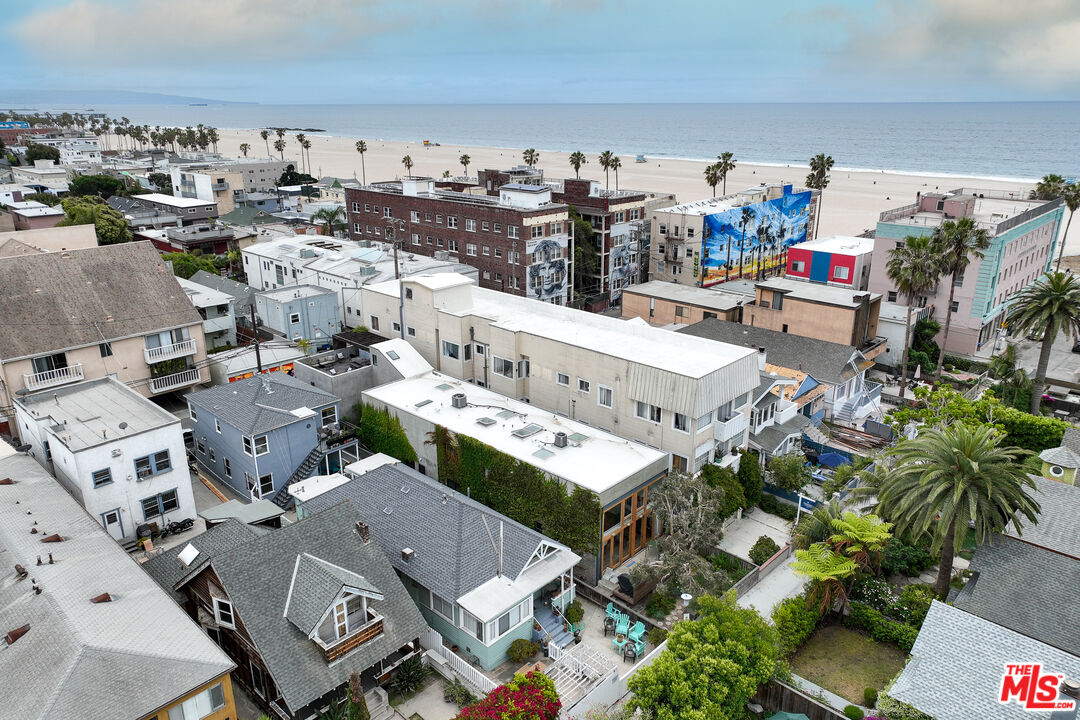This image appears to be a daytime aerial view of a tropical coastal area, likely in Florida. The scene features a beautiful clear blue sky with minimal clouds situated at the top right and left corners of the image. The expansive and serene ocean forms the backdrop, with a faintly visible boat on the top left side. Stretching out in front of the ocean is a white-tan sandy beach, punctuated by numerous palm trees that line the area between the beach and the buildings, as well as some visible on the bottom right of the image. The coastal area is dotted with various buildings and little houses, with some exhibiting vibrant graffiti and art, while others feature patios and multi-story structures up to four stories high. The buildings predominantly showcase colors like white, tan, and a bit of blue. Notably, in the very bottom right-hand corner, there is a red-lettered text reading "the MLS.com."